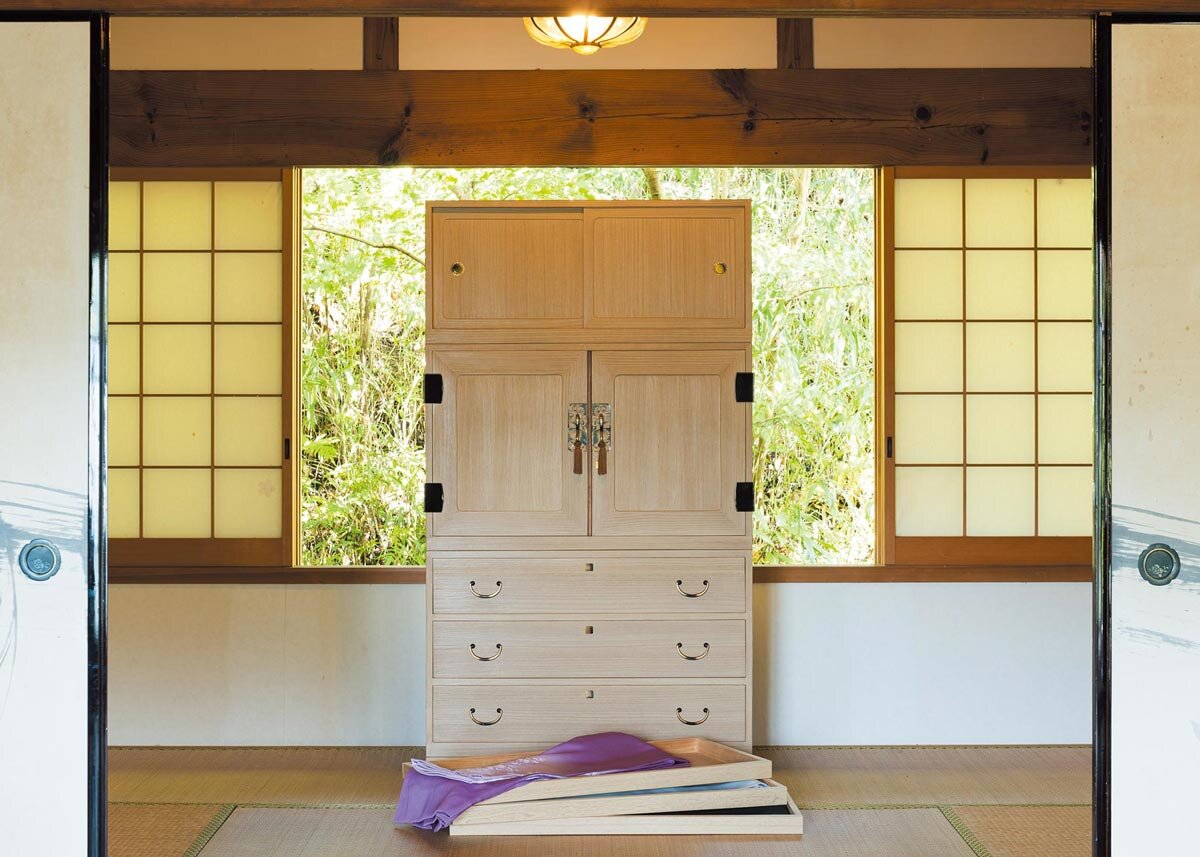The photo showcases a traditional Japanese room featuring tatami mats and a mixture of functional and decorative elements. Central to the room is a large, unbleached wooden cabinet with a distinct, traditional Japanese design. It includes two upper doors that open outward, two lower drawers with what seems to be a silver lock in the middle, and three to four additional long drawers at the bottom.

The room has two sets of sliding doors. The inner sliding doors are outlined in black with beige and light wooden panels, and display blue streaks painted across them. These doors are currently open, revealing an outer set of sliding windows with brown trims and block-like lines, flanked by a white wall with brown wooden floors. Beyond these windows, one can see lush green trees against a bright sky, providing a tranquil view outside.

On the floor, there are three rectangular wooden boxes, each framed in the same light wood as the cabinet. The top box is partially covered by a piece of purple fabric, possibly a towel or clothing, with additional fabrics peeking out from the middle and bottom boxes. A small white light with gold trimming hangs from the ceiling, illuminating the cozy, serene space.